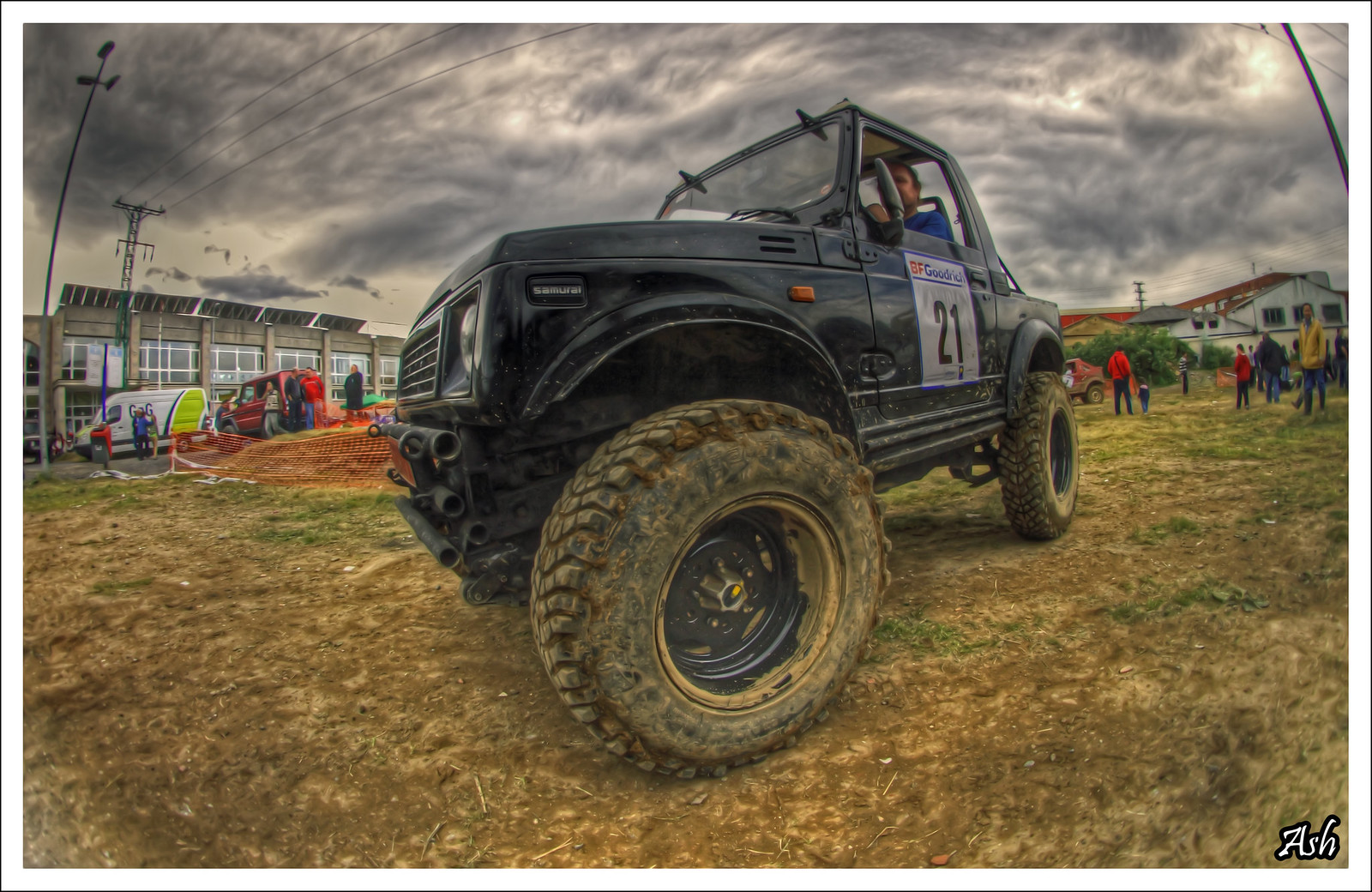This close-up outdoor photo captures a man sitting in the driver's seat of a black Jeep with the number 21 prominently displayed on the door in a white square. He is wearing a blue shirt. The Jeep, which has "BF Goodrich" written on the top, is parked on a muddy dirt area sprinkled with patches of sparse brown and green grass. The scene is set under a very gloomy and cloudy sky, suggesting an impending storm. In the background, there is a bustling crowd, including adults and children. One adult is seen holding a child's hand and walking away from the Jeep. A smaller red Jeep is positioned behind the black one. To the left are several vans parked in front of a building with large glass windows. Additionally, a white house with a red roof is visible among other buildings in the backdrop. The overall atmosphere is one of activity and anticipation against a backdrop of overcast skies and rugged terrain.